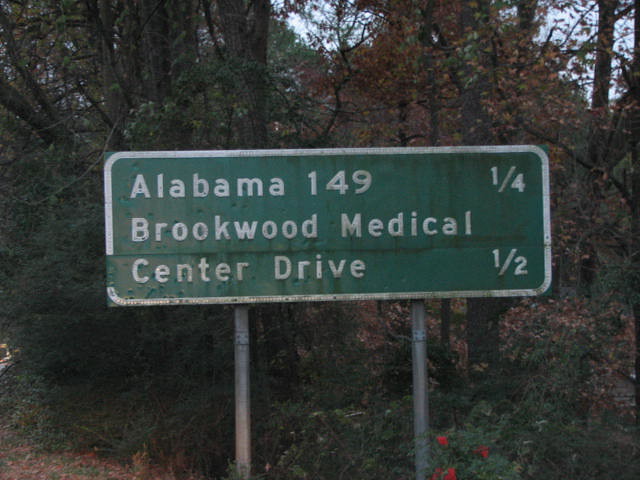This photograph captures a tranquil scene in the woods, likely taken from the side of a road just out of view. The forest features a mix of brown tree trunks and sparse autumn foliage, with hues of orange and pink intermingling among the dried brown leaves on the right-hand side and more vibrant greens on the left. Hints of reddish flowers peek through at the bottom of the image, adding a touch of color to the earthy palette. Dominating the scene is a green rectangular sign with a white border and rounded edges, mounted on two parallel silver metal posts. The sign reads in white text: "Alabama 149," indicating a distance of "1/4" to the right, and "Brickwood Medical Center Drive," with a distance of "1/2" to the right. Above the trees, patches of a cloudy blue sky are visible, providing a serene backdrop to this woodland snapshot.